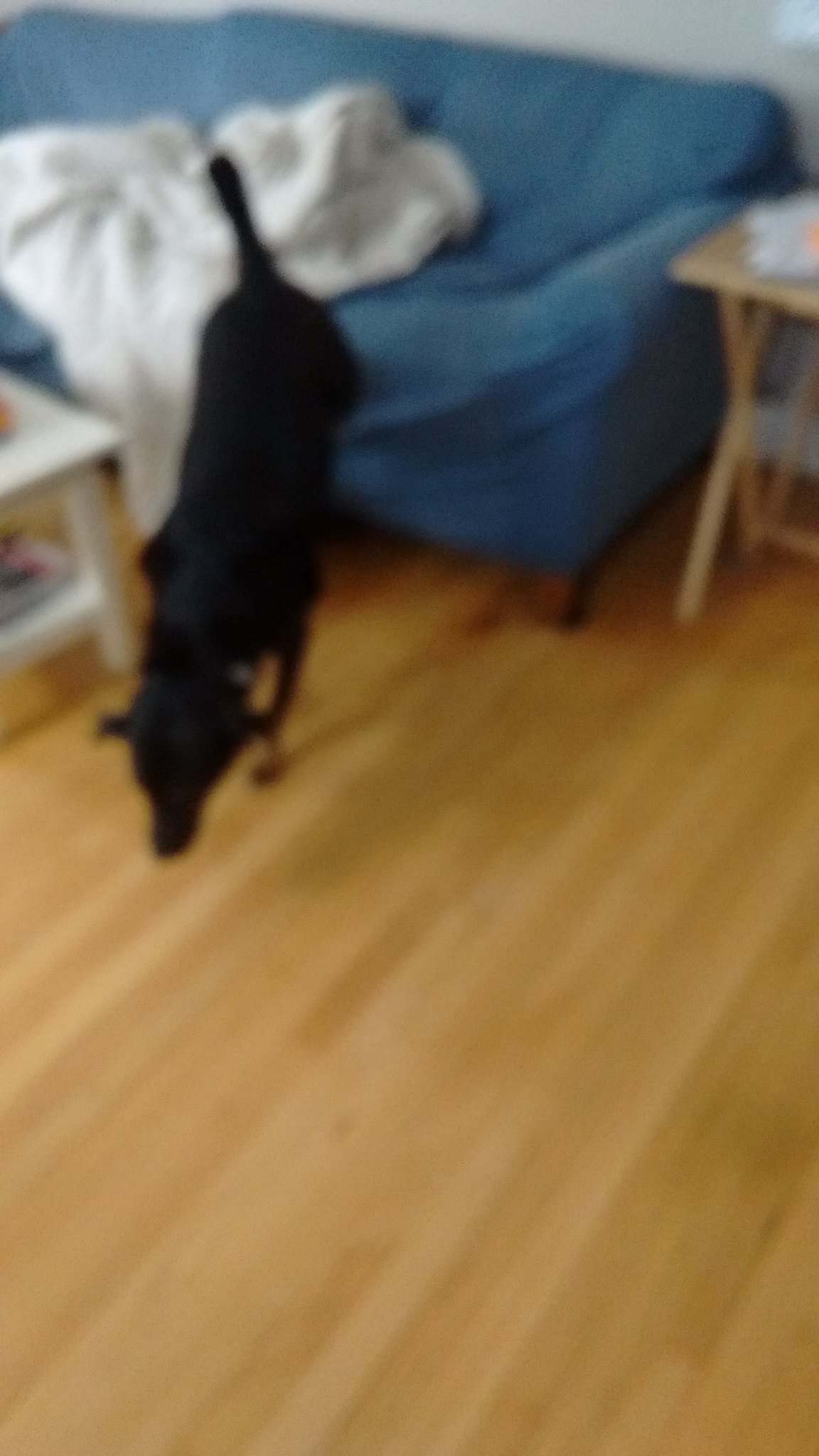The image is a slightly tilted, blurry, first-person perspective photo likely taken with a phone held vertically. It captures a black dog, mid-motion, jumping off a blue couch adorned with a white blanket in the middle. The couch, which has short black legs, is situated against a white wall. In front of the couch, a white coffee table is partially visible, extending out of the frame to the left. To the right of the couch, a wooden stand with folding legs, likely used for placing glasses, holds something white and orange on top. The floors are hardwood, and the overall scene lacks focus, giving it a fuzzy effect where the motion of the dog creates an off-balance, dynamic feel to the image.